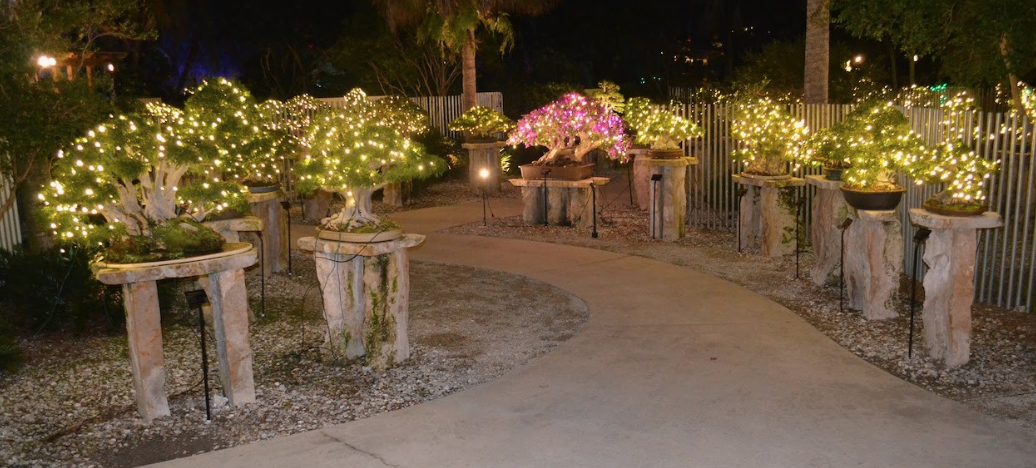This photograph captures a beautifully illuminated bonsai garden at night, possibly situated in a park or private backyard. The garden features a winding cement pathway that begins in the foreground and gently curves to the left, inviting the viewer to take a leisurely stroll. Flanking the path, there are numerous bonsai trees, each meticulously displayed atop stone pedestals. These pedestals, which resemble small circular or oval tables, are about three feet tall, adding to the garden's elegance.

The bonsais, predominantly green, are adorned with bright white LED fairy lights, casting a magical glow on the scene. Among them, one bonsai stands out with its vibrant pink or purple flowers. On closer inspection, there are visible cables extending from the trees, leading out of the frame and enhancing the feeling of a meticulously curated display. Small markers in front of each bonsai provide details about the plant species and their ages, adding an educational touch to the experience.

On the left side of the path, there are two notably larger bonsais. In contrast, the right side hosts six bonsais, maintaining a symmetrical and balanced aesthetic. The backdrop features lofty palm trees silhouetted against the night sky, enhancing the serene atmosphere. The photograph suggests the use of a light source behind the photographer or possibly a camera flash, illuminating the scene delicately. This enchanting setting exudes a sense of tranquility and beckons visitors to explore further into the inviting darkness.